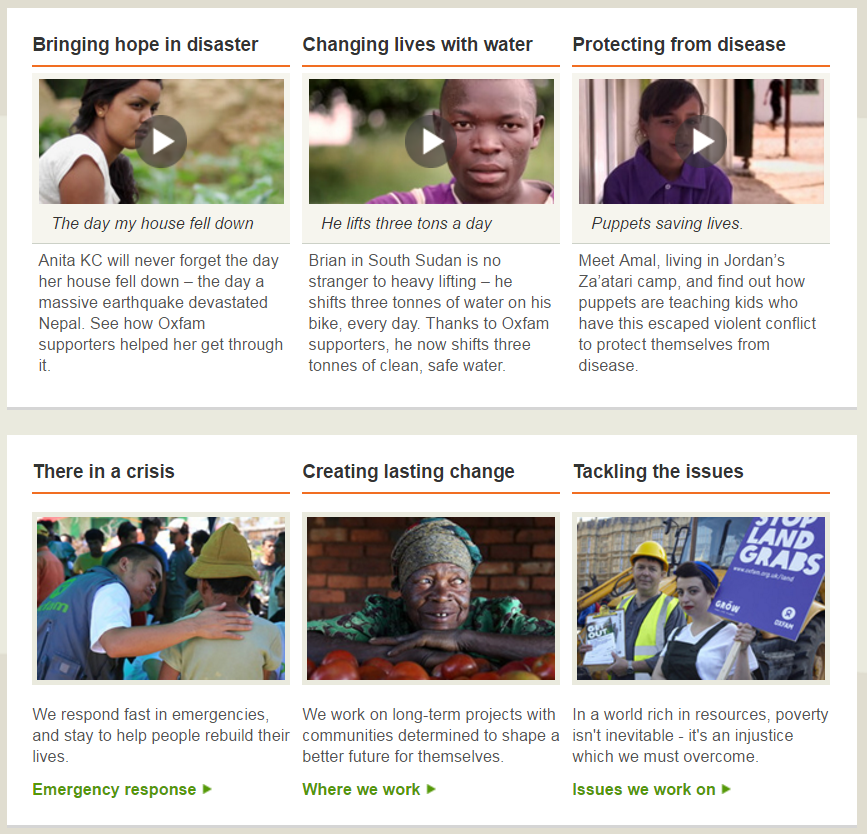The image appears to be a webpage layout showcasing various articles, each encapsulated within a thin, medium-gray border. This border frames the entire image and bisects it horizontally, creating distinct sections above and below.

**Above the Gray Border:**
- **Left Section:** 
  - **Article Title:** "Bringing Hope in Disaster"
  - **Highlight:** An orange bar beneath the title
  - **Visual:** A thumbnail of a video featuring a woman sitting outdoors
  - **Interaction:** A gray circle with a white play button centered on the thumbnail
  - **Quote:** "The day my house fell down"
  - **Description:** Six lines of information about the video content

- **Center Section:** 
  - **Article Title:** "Changing Lives with Water"
  - **Visual:** A thumbnail of a video featuring an African-American man standing outside
  - **Interaction:** A gray circle with a white play button centered on the thumbnail
  - **Quote:** A brief one-line quote from the individual
  - **Description:** Six lines of information about the video content

- **Right Section:**
  - **Article Title:** "Protecting from Disease"
  - **Visual:** A thumbnail of a video featuring a person with black hair and a blue shirt sitting outdoors
  - **Interaction:** A gray circle with a white play button centered on the thumbnail
  - **Quote:** A brief quote from the individual
  - **Description:** Six lines of information about the video content

**Below the Gray Border:**
- **Left Section:**
  - **Article Title:** "They're in Crisis" (Note: "The're" appears to be a typo)
  - **Visual:** A picture of several people standing outside
  - **Description:** Three lines of information
  - **Highlight:** "Emergency Response" in green text

- **Center Section:**
  - **Article Title:** "Creating Lasting Change"
  - **Visual:** An African-American woman leaning her head on what seems to be tomatoes, with a concrete wall in the background
  - **Description:** Three lines of information
  - **Highlight:** "Where We Work" in green text

- **Right Section:**
  - **Article Title:** "Tackling the Issues"
  - **Visual:** A picture of people holding up a sign outdoors
  - **Description:** Three lines of information
  - **Highlight:** "Issues We Work On" in green text

This layout effectively divides the information into multiple sections, with each article accompanied by a visual representation and concise descriptive text, making it easier for viewers to engage with the content.